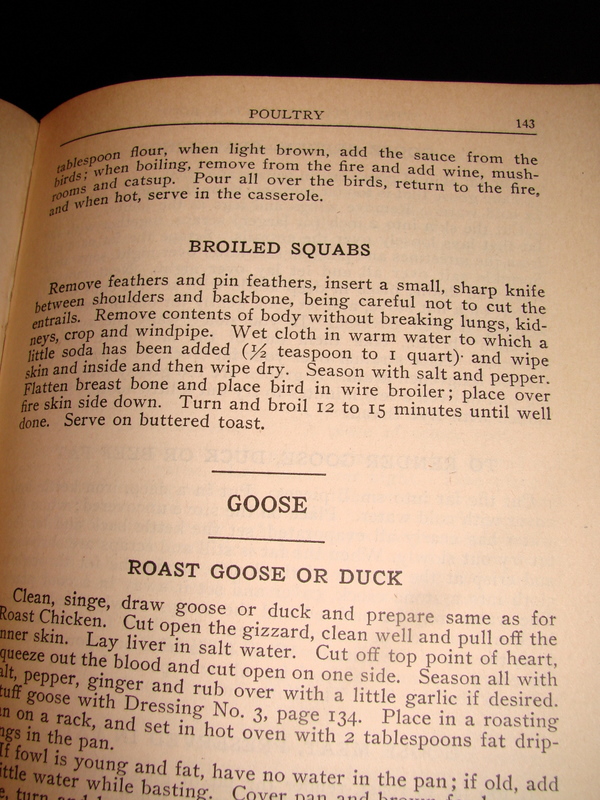The image depicts a close-up page from a cookbook, specifically page 143, with a tan-colored background and black text. At the top of the page, the heading "Poultry" is prominently displayed, followed by instructions and recipes. The segments covered include "Broiled Squabs" and "Goose." 

In the "Broiled Squabs" section, detailed steps instruct on removing feathers, pin feathers, and various parts carefully, followed by cleaning with a solution of warm water and soda, seasoning with salt and pepper, and broiling the bird until well done. It ends with a serving suggestion of placing the broiled squabs on buttered toast.

The section labeled "Goose" specifically addresses preparations for both "Roast Goose or Duck." Instructions are provided on cleaning, singeing, and preparing the bird similar to roast chicken, followed by further cooking directions that include adding a sauce made from wine, mushrooms, and ketchup, returning the dish to the fire, and serving hot in a casserole.